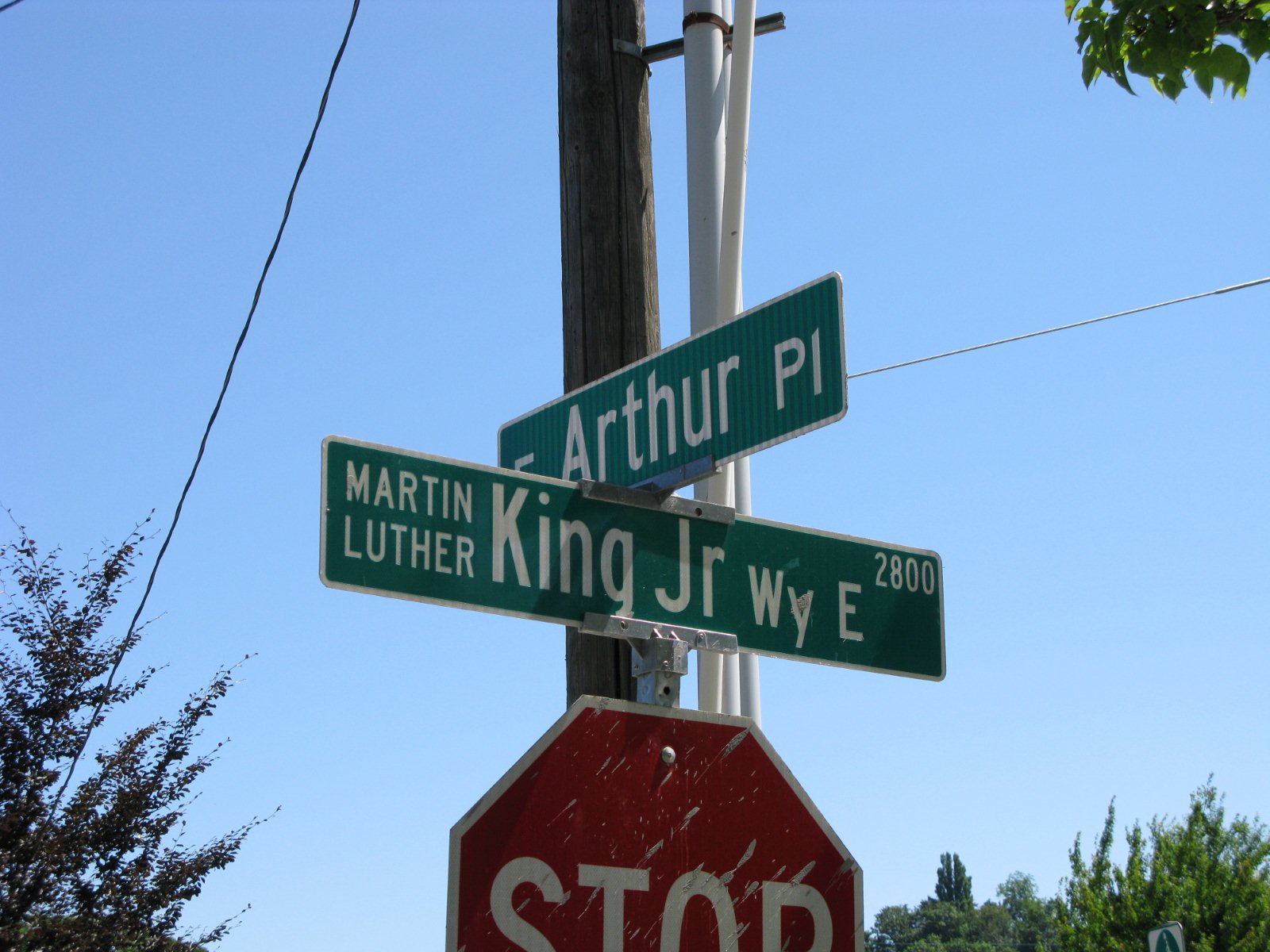This image is a detailed color photograph taken from below, slightly angled upward, capturing a stop sign and two intersecting street signs on a clear, bright, sunny day with a cloudless blue sky. The main focus is on the signage, where the green street signs with white lettering are positioned perpendicularly at a 90-degree angle atop a pole. The top sign reads "Arthur P.L." and the bottom sign indicates "Martin Luther King Jr. Way E, 2800." Below these signs, a red stop sign with white lettering shows noticeable diagonal scratching. The wooden pole, brown in color, extends vertically through the image, accompanied by a connected white pole. Multiple cables crisscross the scene, with one diagonal on the left side of the image and another extending straight to the right. Surrounding the signage are trees with varying shades of green, visible in the bottom left corner, bottom right corner, and top right corner of the image. The photograph captures the vibrant essence of the intersection, highlighting both the signage and the natural elements under a pristine sky.